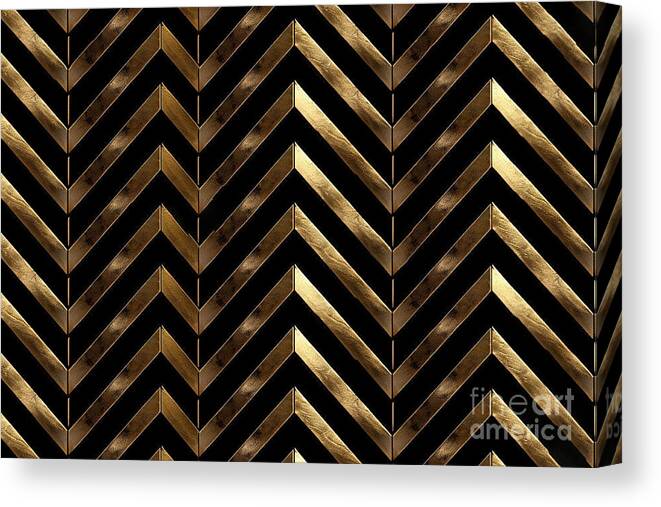The image features a textured piece of art in a landscape orientation, showcasing a vivid black and gold chevron pattern. This pattern, composed of wood beams with a golden metallic texture and a matte black finish, creates an intriguing 3D effect where sections appear to pop out while others seem recessed. The chevron design is arranged in columns, giving the impression of three distinct vertical sections. The intricate pattern not only adorns the front but also wraps around the sides, enhancing the dimensional effect. The backdrop of the image is black, making the gold elements glisten prominently. A fine light watermark reading "Fine Art America" is visible in the bottom right corner.